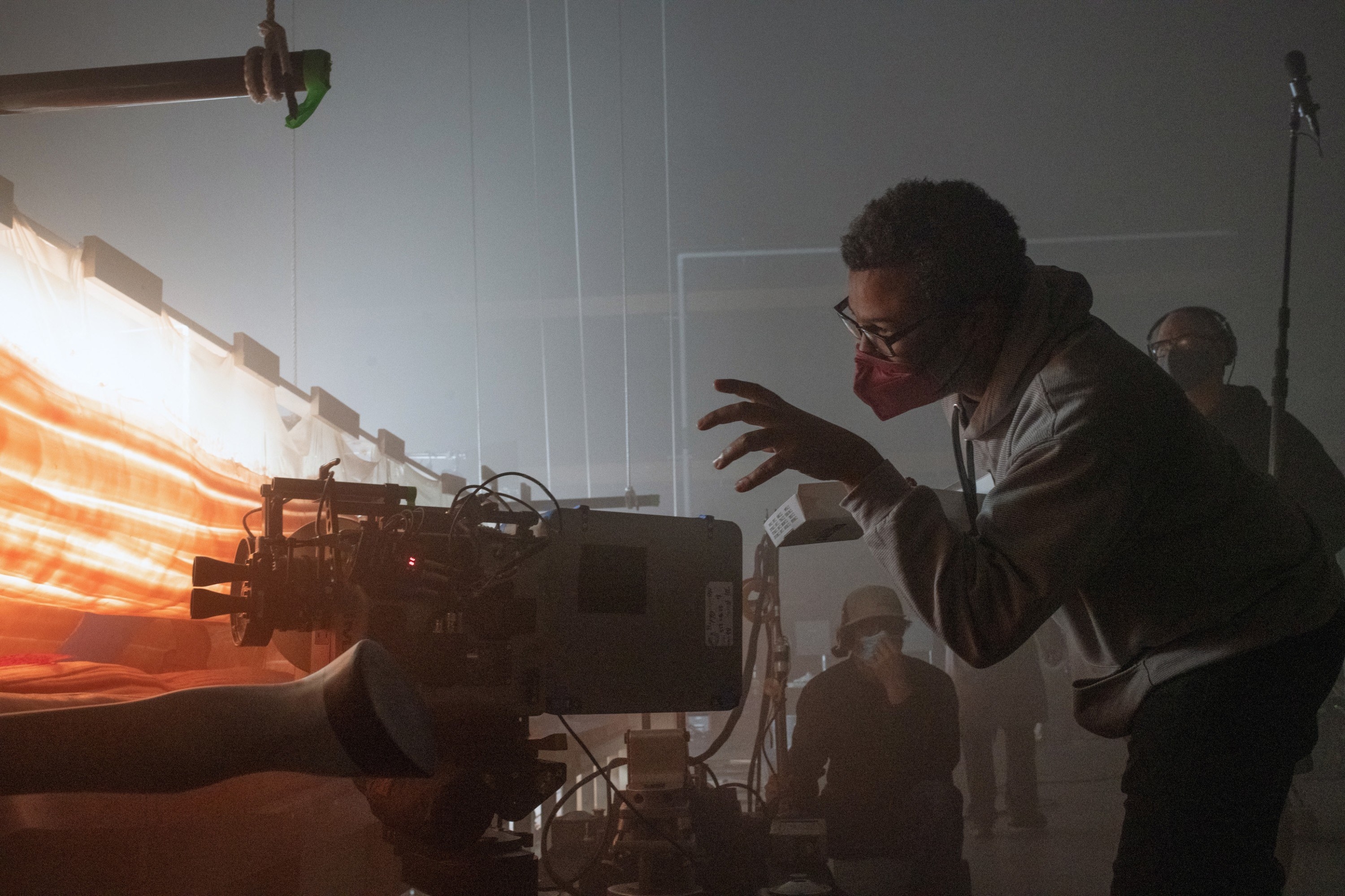In this photograph, we observe a bustling behind-the-scenes moment from what appears to be a movie set, captured in landscape orientation. The scene is set in a somewhat smokey and hazy atmosphere, hinting at a production environment during the COVID-19 pandemic, as evidenced by the masks worn by all individuals present.

On the right side, a person of African American descent with black hair and a red mask stands out, seemingly directing or orchestrating the scene. This individual is dressed in a gray hoodie and jeans, extending their left hand toward a large, intricate camera equipped with various lenses and wires. Close by, a man kneels with his hand on his mask.

To the left, an unusual visual element—a horse's hoof—is visible, jutting into the scene, adding an almost surreal dimension against the otherwise realistic set. Behind the central figure, another man, possibly an assistant, holds a microphone. There are also several headsets and hats seen amidst the crew members, enhancing the professional setup.

The backdrop includes a distant wall, illuminated lighting fixtures on the far left, and numerous ropes or wires hanging from above, securing objects and contributing to an overall production-studio ambiance. Additionally, some sort of plastic wall seems to be part of the set, further indicating that this image captures a meticulously arranged moment of filmmaking.